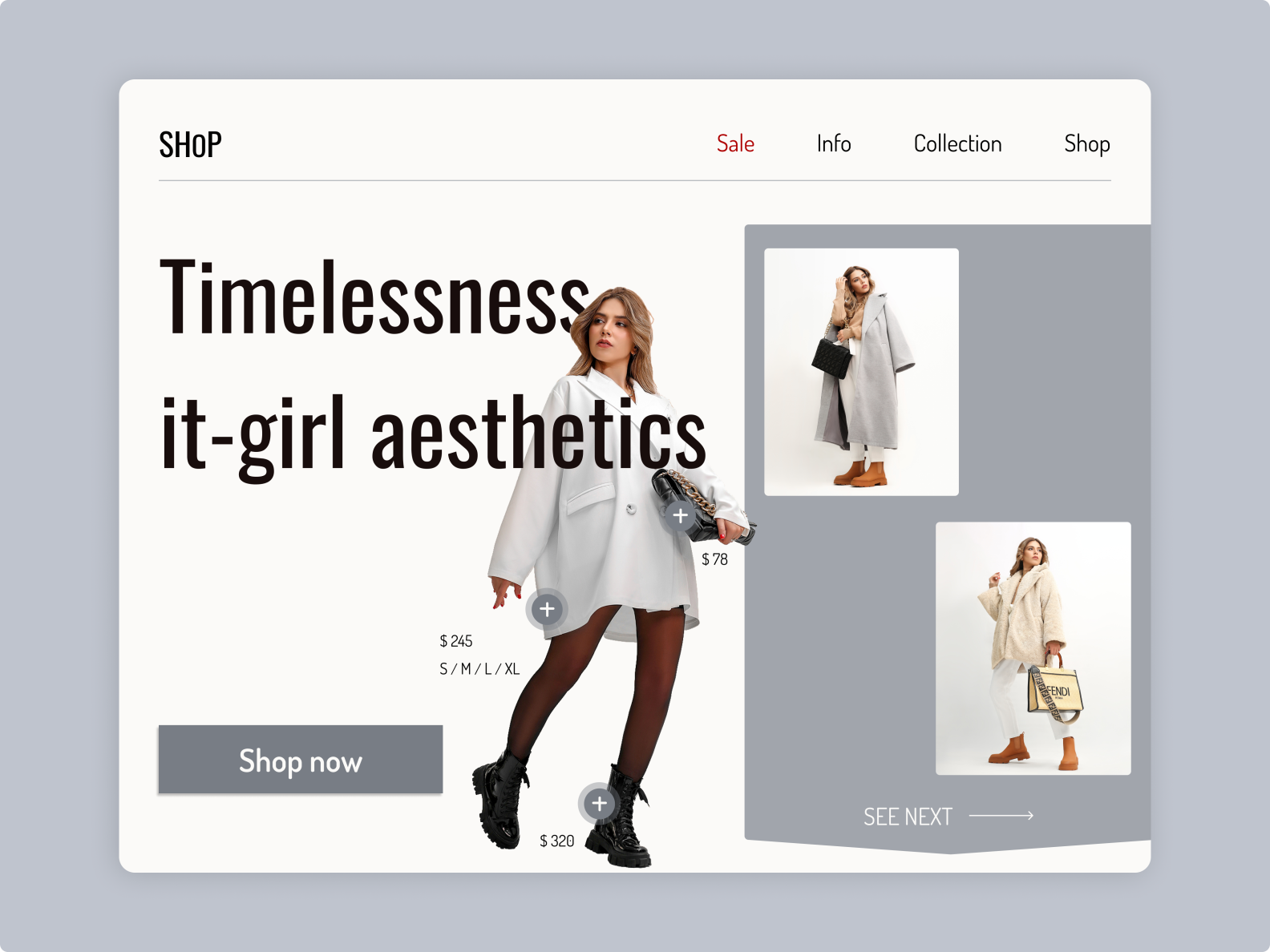The image appears to be a mock-up of a modern e-commerce website with a minimalist design. The central focus is a white panel with subtle drop shadows, positioned against a light gray background. At the top of this panel is a navigation menu, accompanied by a logo in the upper left-hand corner. The logo is styled in all uppercase letters, but notably, the "O" is smaller than the other letters and less tall, creating a distinctive look. A thin gray line runs horizontally beneath the logo, spanning the entire width of the panel, which features rounded corners.

The menu offers four options: "Sale" in red, followed by "Info," "Collection," and "Shop." Below this, a model takes center stage. She is dressed in an oversized, double-breasted white shirt or jacket, the large size obscuring any other clothing she may be wearing underneath. Her ensemble is completed with black boots. The model has blonde hair and holds a purse or bag. Alongside this, the text reads: "Timelessness. It's Girl Aesthetics. $245," indicating the pricing for the shirt/jacket, available in sizes Small, Medium, Large, and XL. Notably, there are plus icons, one over the shirt/jacket, and another over the purse, which is priced at $78. A gray "Shop Now" button is located towards the lower left of the model.

To the right of the main image is a gray panel featuring two staggered photographs, positioned in the upper left and lower right corners. These photos show the same model. In the first image, she carries a briefcase and wears an extremely oversized gray jacket along with brown boots. In the second photo, she dons the same brown boots paired with white pants, a Fendi bag, and a fluffy, oversized white jacket. The panel concludes with the text “See Next,” suggesting further browsing options.